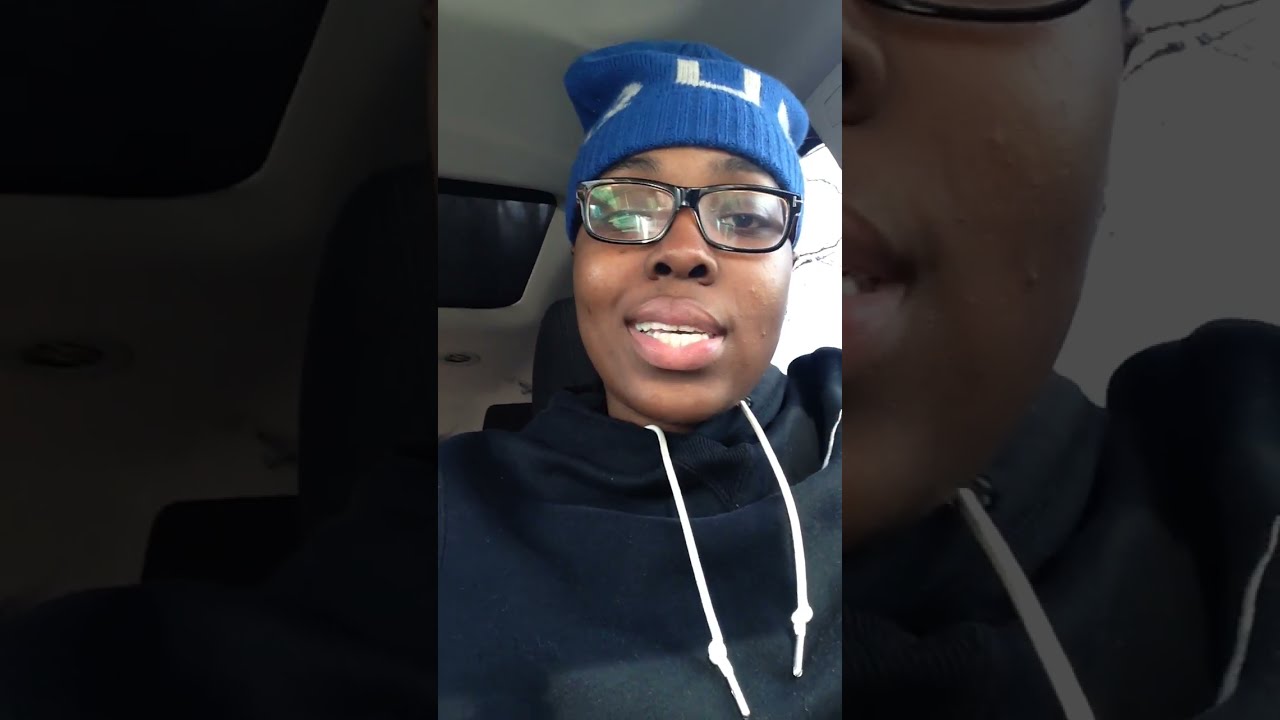A close-up image captures a black woman in a car, looking directly at the camera with a concerned expression. She has neatly styled, rectangular-shaped eyebrows and dimples, and is wearing black, thick-rimmed glasses that reflect light from both lenses. Her mouth is closed tightly, with her top lip slightly overlapping her bottom lip. She is dressed in a dark navy hoodie featuring white strings hanging down, and a small white button is visible near the bottom of the hoodie. Her head is covered by a blue knit beanie with a white strap on top. The background reveals the inside of a vehicle, with a window and ceiling visible, and light entering from the side.